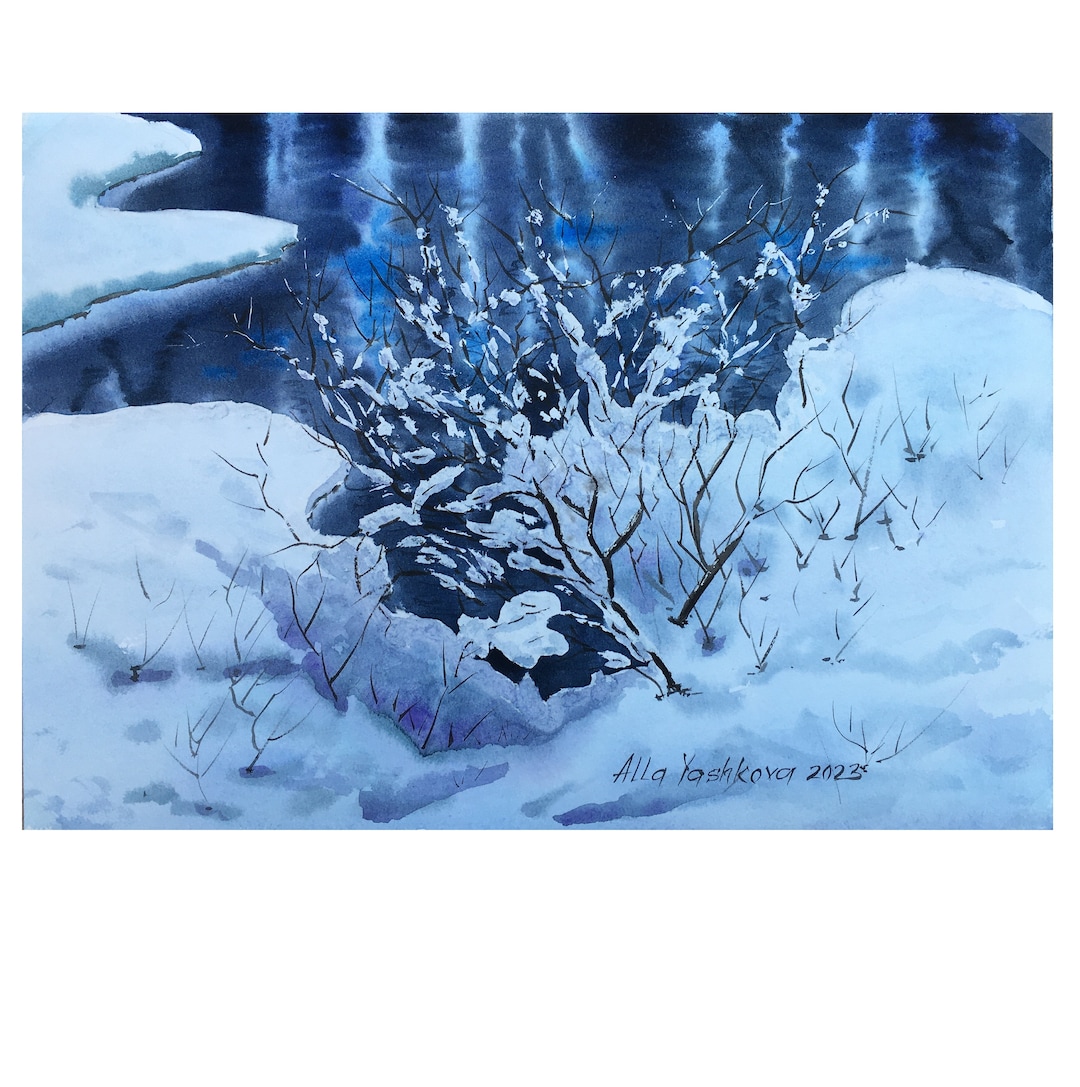The image is a watercolor painting of a serene snow-covered scene, signed "Allen Yashkoba, 2023" in a handwritten style at the bottom. The composition is dominated by shades of blue and white, creating a soothing winter atmosphere. In the foreground, a large expanse of snow is punctuated by a central shrub with barren, black branches delicately adorned with clumps of snow. Surrounding it are smaller shrubs and sticks, similarly leafless and dusted with snow. To the left, another patch of snow protrudes, adding depth to the snowy landscape. The upper portion of the image features a pool of water, likely partially frozen, with blue and white reflections that suggest an icy surface. The overall effect is a tranquil depiction of a snowy outdoor scene, artistically capturing the quiet beauty of winter.